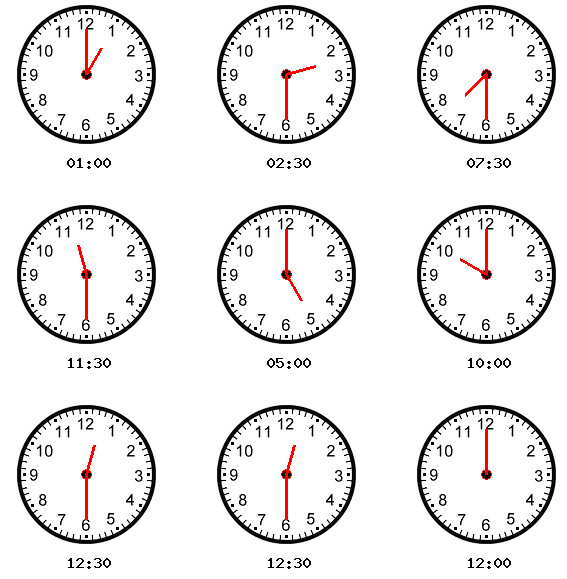The image features an array of nine analog clocks meticulously arranged in a 3x3 grid against a pristine white background. Each clock is circular with a white face, marked with standard black numerals from 1 to 12, and outlined in black. The clock hands are a striking red, providing a vivid contrast. Below every clock, the displayed time is clearly indicated in black numerals. Starting from the top-left corner and moving across the row, the clocks display the times: 1:00, 2:30, and 7:30. In the middle row, the times are: 11:30, 5:00, and 10:00. In the bottom row, the times are: 12:30, 12:30, and finally 12:00. There are no additional elements in the image, highlighting the simplicity and clarity of the scene.